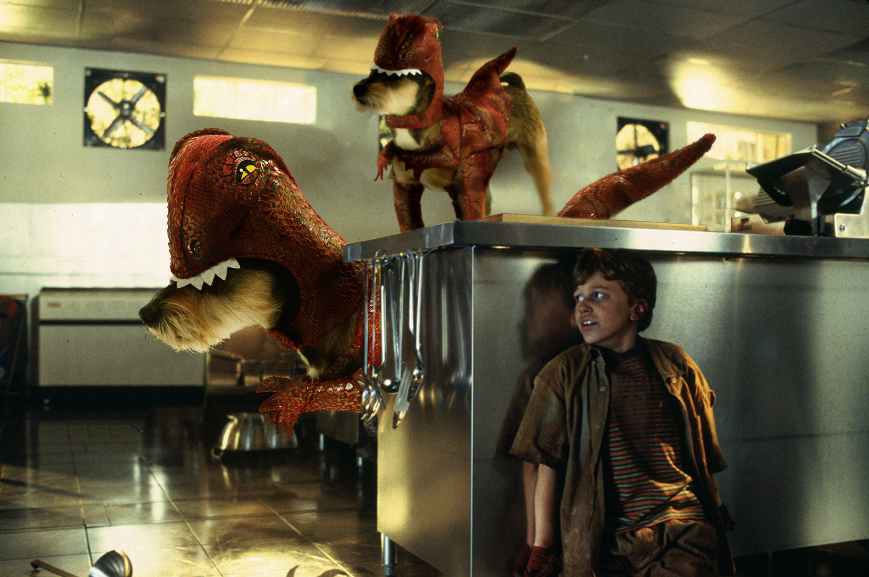In an industrial kitchen setting, a boy clad in a striped red and blue shirt with a pale brown unbuttoned button-up over it, sits scared on the ground beside a stainless steel table. The table, set against a light green wall with stainless steel cabinets behind and a plain white wall, has large utensils hanging from its left side. The boy, who seems to be part of a scene reminiscent of Jurassic Park, gazes fearfully to his right. On the opposite side of the table, two brown dogs dressed in red Tyrannosaurus Rex costumes add a peculiar twist to the scene. The room is dimly lit with sunlight streaming in through small, narrow windows on the opposing wall.